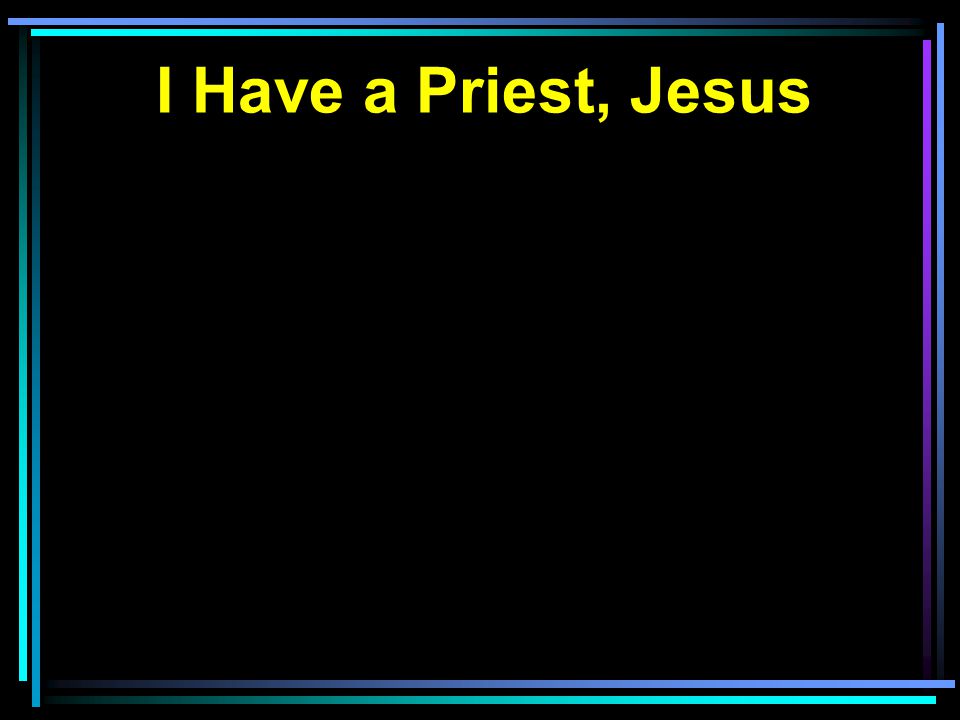The image features a predominantly black background with a two-line border that encompasses a bluish to purple hue, displaying shades of blue, teal, and purple in varying intensities. The border is uniformly colored except on the right side, where the bottom line is purple instead of light blue. Just below the top border, the image showcases bold, centered, and large yellow text that reads, "I have a priest, Jesus." The font is formal and neat, and there are no additional elements or text within the image apart from the yellow inscription at the top. The central expanse remains a stark, solid black, emphasizing the simplicity and focus on the highlighted text.